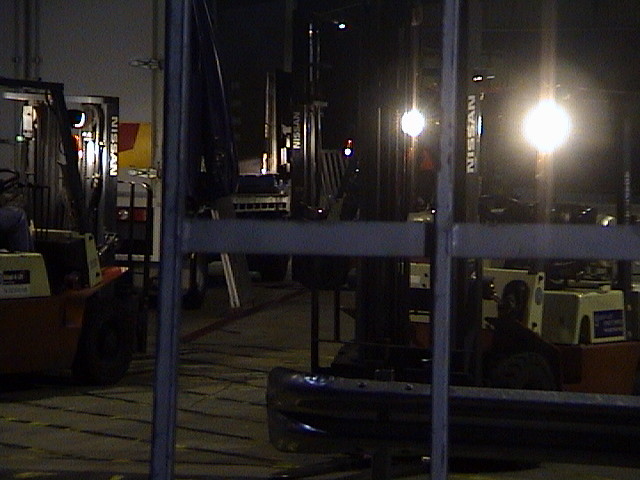The photograph captures the interior of a large, industrial building, likely a warehouse or factory, under low light conditions. The scene features an array of construction equipment, including several forklifts prominently positioned on a gray cement surface marked with black and yellow safety stripes. Details on one of the forklifts, which is orange, yellow, and black, reveal the brand "Nissan" written in white sideways letters. 

The image is predominantly dark, with illumination coming from two bright white light sources at the front, possibly headlights from vehicles such as trucks or forklifts. Two tall, dark blue metal poles extend vertically from the floor to the ceiling, positioned slightly off-center, with a horizontal navy blue metal beam connecting them midway. In the back right of the image, light shines onto a steel structure that seems to incorporate glass windows, adding to the industrial aesthetic of the space. The overall setting conveys a sense of nighttime operations within the warehouse, highlighting the metallic infrastructure and the strategic layout of machinery and equipment.